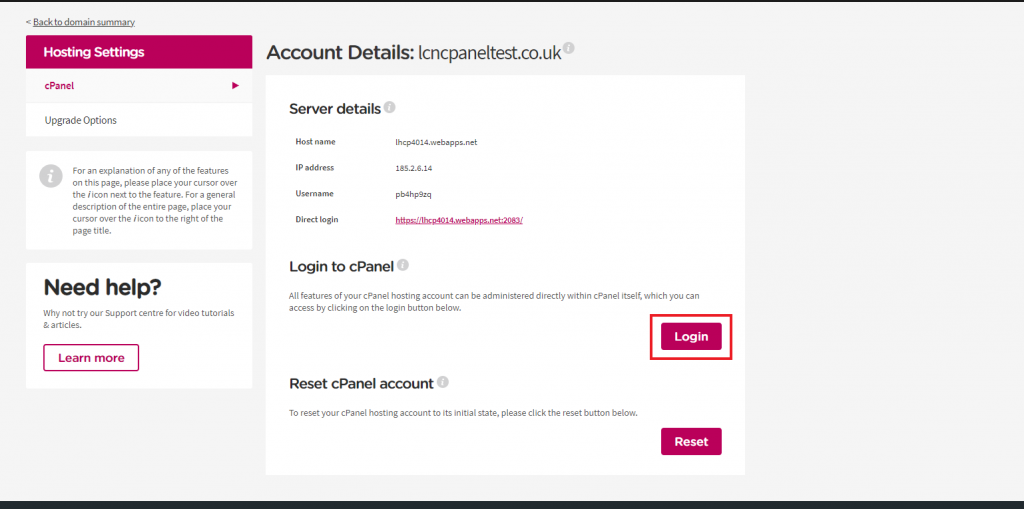Screenshot of a computer screen showcasing the hosting settings of a cPanel interface. 

In the top-left corner, there is a link labeled "Back to Domain Summary." Below this is a bold red heading titled "Hosting Settings." An arrow pointing towards "cPanel" is displayed beneath the heading. Following this, there are "Upgrade Options" and an informational box with an eye icon. The box reads: "For an explanation of any of the features on this page, please place your cursor over the eye icon next to the feature. For a general description of the entire page, place your cursor over the eye icon to the right of the page title."

Further down, there's a highlighted section with bold text stating, "Need Help?" and suggests visiting their Support Center for video tutorials and articles. A red-outlined button labeled "Learn More" is also visible.

Under "Account Details," it mentions the domain "ICNCpaneltst.co.uk" along with an eye icon for more information. "Server Details" are provided, including the hostname "IHCP4014.web.apps.net," IP address "185.2.6.14," and a slightly blurry username that appears to be "PB4HP2SQ."

The interface includes a section for "Direct Login," explaining that all cPanel hosting account features can be accessed by clicking the "Login to cPanel" button below. There's also an option to "Reset cPanel Account," advising users to click the "Reset" button to revert the account to its initial state.